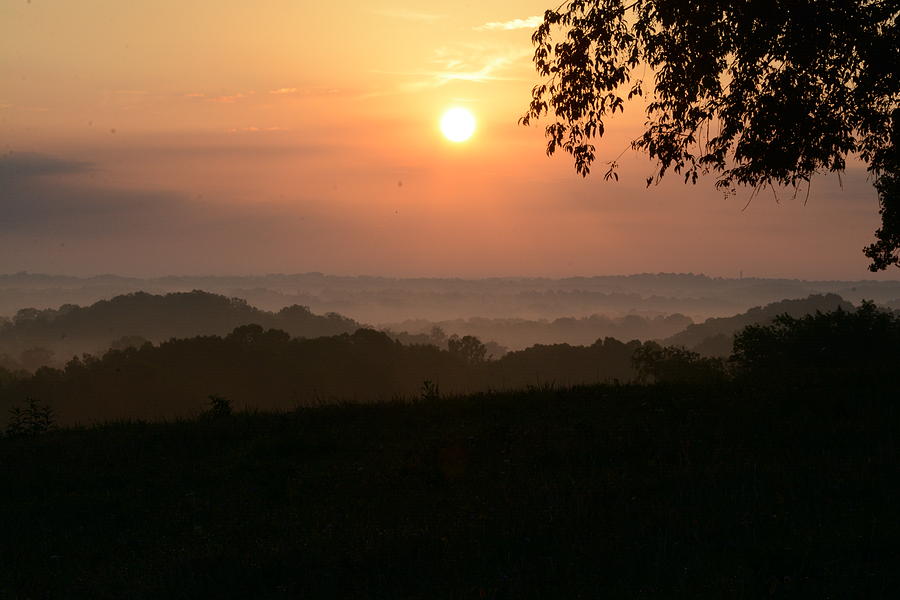The photograph captures a serene late afternoon sunset from atop a hill, enveloping the landscape in a soothing blend of warm colors. The sun, almost white with a bright yellow halo, sits low in the sky, diffusing a light peachy hue that transitions to pink and then to gray toward the horizon. Silhouetted branches and leaves from a large tree occupy the upper right corner, adding a contemplative element to the scene. Below, rows of trees stretch across rolling hills cloaked in a delicate, foggy mist, shifting from green to gray as they recede into the distance. The grassy area at the bottom of the image, dotted with bushes, appears greener than the rest, bringing a fresh contrast to the overall warm and inspirational ambiance. The sky, painted with orange and yellow hues, carries a few dim, yellow-tinted clouds that blend seamlessly into the tranquil scenery, creating a sense of calm and inspiration, perfect for reflecting on the day's end.